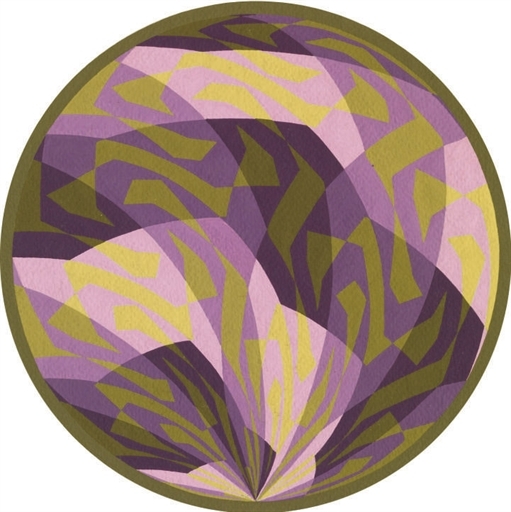The image is a photograph of a circular piece of abstract modern art. The perfect circle is framed by a dark bronze or golden olive-colored rim. Inside, the design features a vibrant, geometric composition with varying shades of purple, ranging from light lilac and lavender to medium and dark plum. Interspersed among the purple sections are irregular, geometric patches and splotches of a lighter olive or gold color, forming various shapes like squares and rectangles. The texture suggests it could be watercolor on paper, although it might also be computer-generated. The overall artwork is visually appealing and measures approximately six inches in diameter. There is no text, date, or artist's signature visible on the piece.